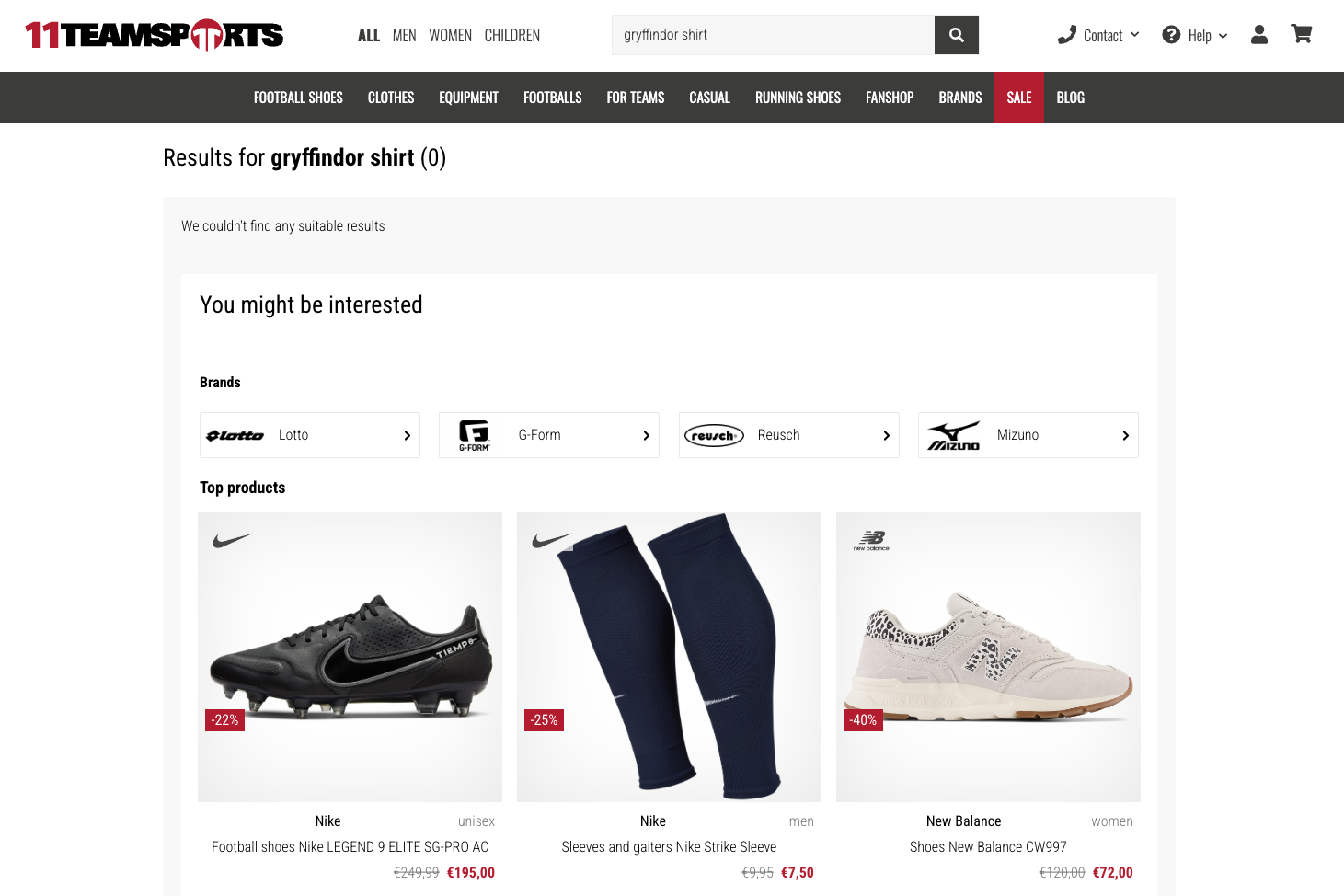The image is a detailed screenshot from a sports apparel website named "11 Team Sports," prominently displayed in the upper left corner. At the top, the navigation bar features several buttons labeled "All," "Men," "Women," and "Children," along with a central search bar where the term "Gryffindor shirt" has been entered. Adjacent to the search bar are links for "Contact" and "Help," in addition to a profile icon and a shopping cart button.

Beneath this main navigation, there are multiple category tabs: "Football Shoes," "Clothes," "Equipment," "Footballs," "4 Teams," "Casual," "Running Shoes," "Fanshop," "Brands," "Sale," and "Blog."

On the left side of the webpage, a section labeled "Results for Gryffindor Shirt 0" indicates that no matching products were found. A message below this states, "We couldn't find any suitable results you might be interested in," followed by three product suggestions: "Nike Football Shoes," "Nike Legend 9 Elite," and a pair of "Nike Sleeves and Gators." Additionally, "New Balance Shoes" featuring the "New Balance CW997" model is displayed.